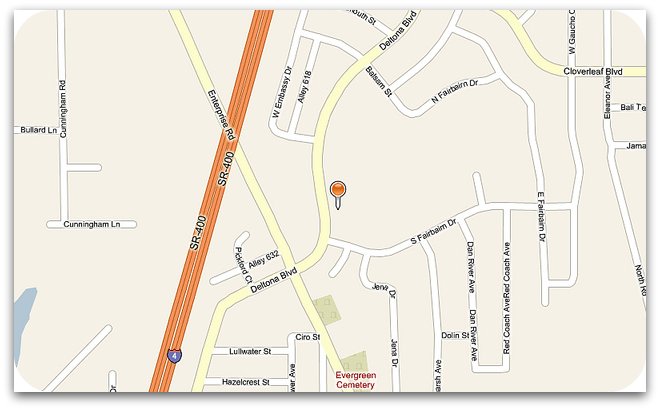This image shows a detailed section of a map primarily rendered in light beige tones. Distinguishing the major routes, the SR 400 highway runs through the left side of the frame, depicted in a darker orange hue, contrasting with the pale yellow of other major streets. Minor streets appear in white, weaving intricate pathways across the map. 

At the center of this detailed section, an orange pen marks a location, though it remains unlabeled and provides no address. The map features labels for several streets, like Bullard Lane, Cunningham Road, Cunningham Lane, and Cloverleaf Boulevard, which meander predominantly across the right and lower center portions of the image. Distinctively, an "Evergreen Cemetery" is highlighted in red near the bottom center, serving as one of the few identifiable landmarks. 

However, the map lacks any indicators of the overarching city or state in which this area is located, adding a layer of ambiguity to its geographic context.